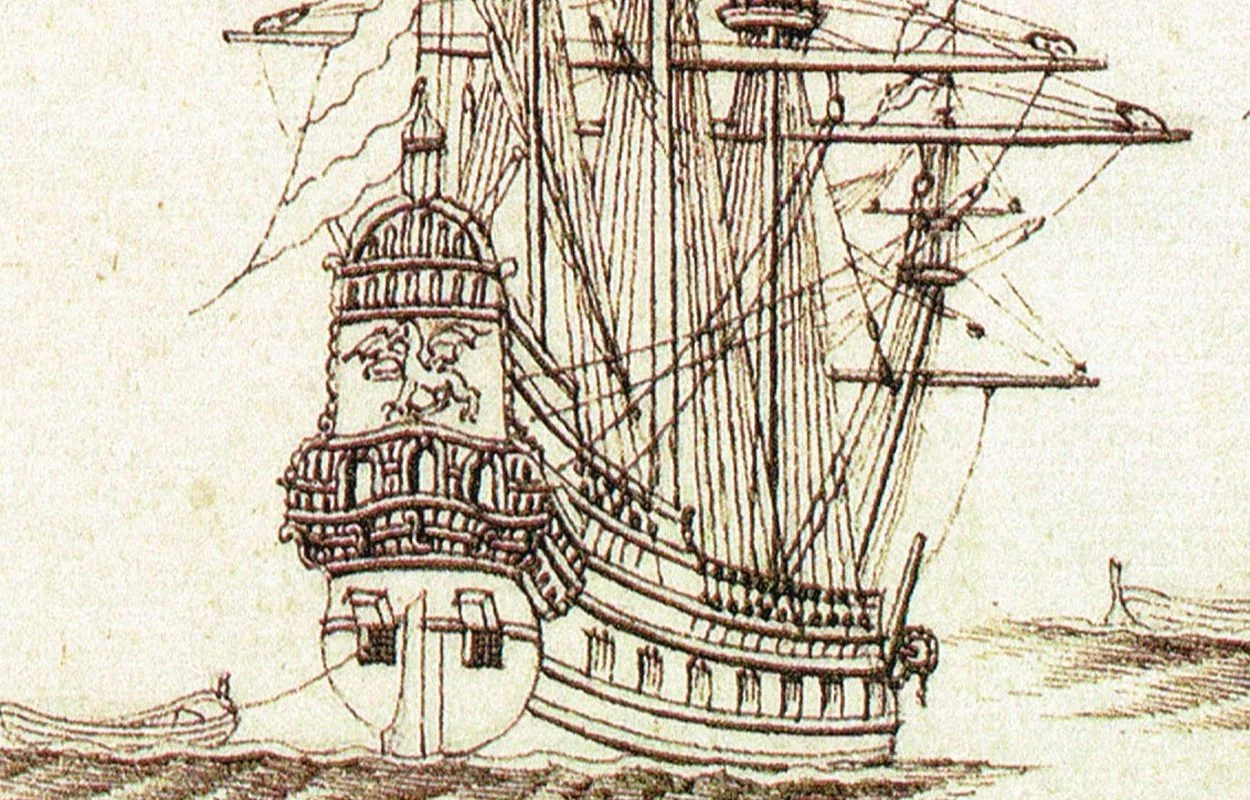The drawing showcases a large, aged Viking ship with a striking, intricate design. Rendered in dark brown and black tones on a yellowed surface, the illustration exudes an air of antiquity. The ship is depicted in rough waters, advancing towards the viewer. Prominently featured on the ship’s prow is a large shield-like crest adorned with a flying horse-like creature, accompanied by decorative carvings and arches. Numerous masts and extensive rigging hint at the majestic sails that would have adorned the vessel, though none are currently unfurled. Along the base and on the front, several windows are visible. A small rowboat, tethered to the ship’s left side, floats amid the waves. In the distant background, another ship appears, possibly in distress, without its masts visible. This detailed and carefully executed pencil drawing, possibly dating from the 1800s or 1900s, captures the essence of a historic seafaring vessel with precision and care.